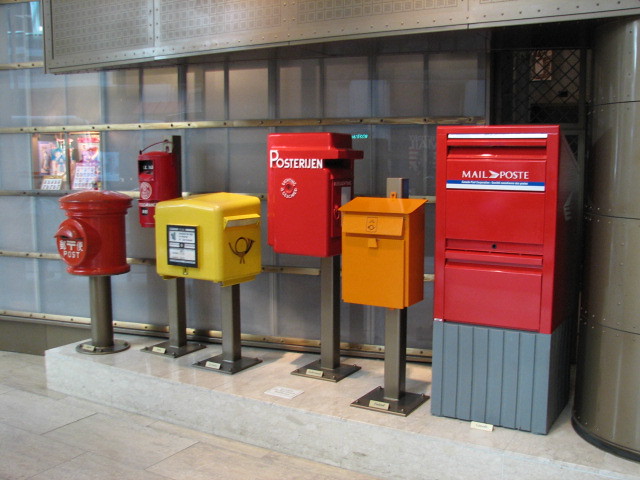This image is a vibrant color photograph capturing the exterior of a European post office setting, distinguished by its clean, ceramic tile flooring and raised white tile platform. Positioned neatly in front of a curved, steel gray building with windows, there are six distinct mailboxes, each varying in shape and size. Beginning from the left, the first mailbox, small and red, somewhat resembles a fire hydrant. Next to it stands a taller, cylindrical red mailbox. The third in line is a large, square yellow box. The fourth mailbox bears the inscription "Posterium" and is also red. An orange mailbox follows, designed to be opened from the top, resembling a box. The line concludes with a larger red mailbox inscribed with "P-O-S-T-E." Each mailbox is mounted on a concrete ledge, and small plaques are visible on the ground beside them, suggesting this array might be part of a display, possibly within a museum-like setting. The meticulous arrangement and pristine surrounding imply an organized and curated presentation, highlighting the variety and evolution of postal mailboxes.